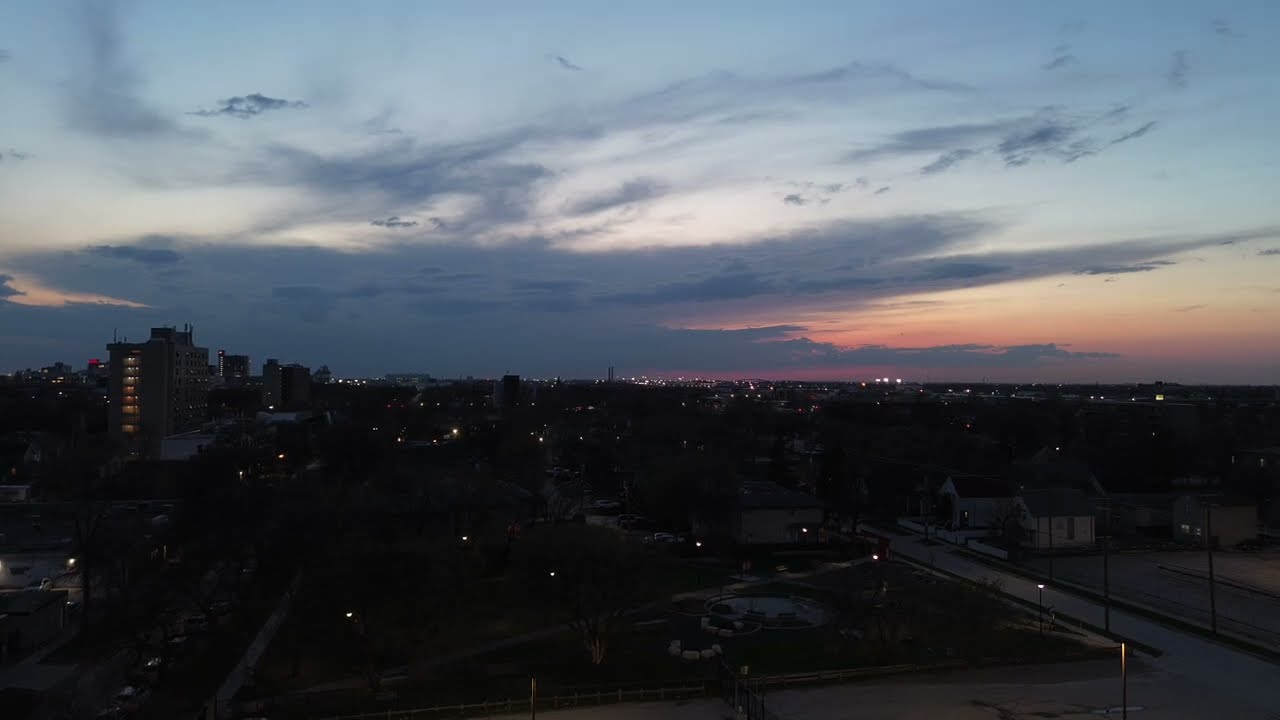In this image, we're presented with a captivating cityscape set at dusk. The setting sun bathes the horizon in a warm palette of red, orange, and yellow, while the remainder of the sky above transitions to a serene light blue. Wispy clouds roll in from the center-left, their edges tinged with the final hues of day. The foreground is dominated by a darkened residential area, punctuated only by the soft glow of numerous street lamps scattered throughout. To the right, an outline of a large building with a notably darker roof is just discernible, suggesting the boundary of this tranquil urban scene. On the left-hand side, taller multi-story buildings rise, some of them shining with illuminated windows. These structures, possibly apartment complexes or business buildings, provide a vertical contrast to the otherwise low-lying surrounding houses. Nestled in the bottom center of the image is a green park area, a small oasis outlined by the faint luminescence of the city lights. Overall, the image captures a peaceful transition from day to night, highlighted by the interplay of natural and artificial light.